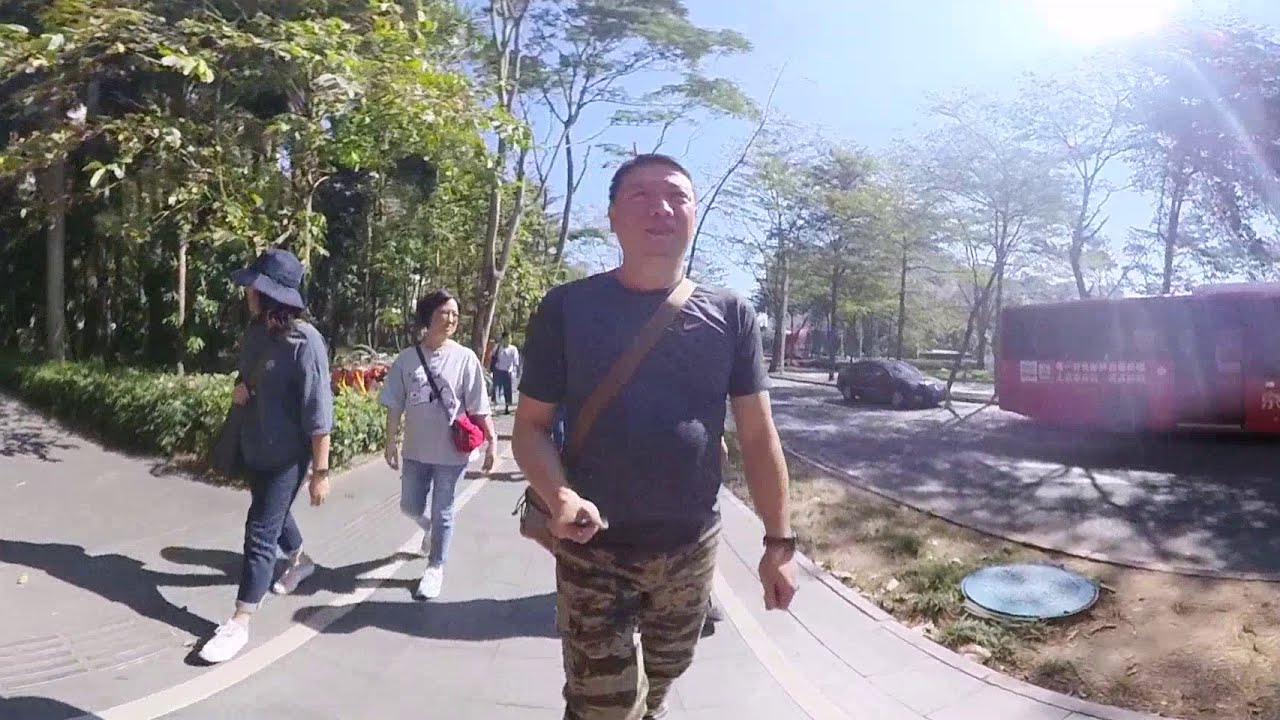In the image, an Asian man is walking down the center of a footpath next to a busy road, wearing a blue t-shirt and camouflage pants. He has a bag draped across his shoulder down to his hip and is holding a selfie stick that’s capturing the scene. His left leg appears thinner, possibly indicating an artificial limb. To his left, there are two women walking close by. The first woman is wearing a light pink or gray shirt with light blue pants and a red bag with a black strap slung over her opposite shoulder. The second woman is slightly ahead, dressed in a dark blue long-sleeved shirt, matching pants, and a wide-brimmed hat, and has a brown bag across her shoulder. In the background, between the man and the first woman, another person in a white shirt is seen walking forward. The scene is outdoors during the daytime under bright blue skies. To the right of the group, there is a red bus and a parked sedan on a two-way road. The left side of the image shows a branching pathway and is lined with lush green trees and shrubs, enhancing the vibrant atmosphere of the setting.